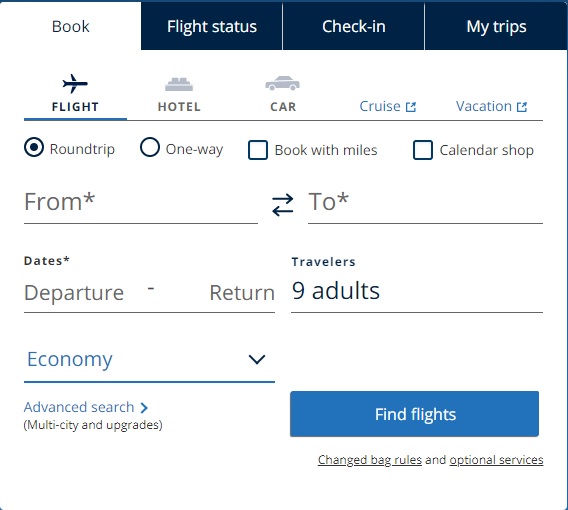Here is a cleaned-up and detailed caption for the screenshot of the chart:

---

This is a screenshot of a chart from a flight itinerary website, depicting the "Book" section. The chart displays four primary tabs at the top: "Book," "Flight Status," "Check-in," and "My Trips." The "Book" tab is currently selected and highlighted with a white background, while the other tabs have a blue background. Within the "Book" section, there are sub-tabs labeled "Flight," "Hotel," and "Car," followed by options for "Cruise" and "Vacation." The "Flight" sub-tab is underlined, indicating that the details shown pertain specifically to flights.

Below the "Flight" icon, there are two selectable bubbles labeled "Round Trip" and "One Way," alongside checkboxes for "Book with miles" and "Calendar shop," aligned in a row. The "Round Trip" option is selected. The chart includes input fields for "From" and "To" locations, both of which are currently empty. Additionally, date fields are also empty. The traveler information indicates "9 adults," and the flight selection is set to "Economy."

At the bottom of this section, there is an "Advanced Search" option offering "Multi-city" and "Upgrades." Finally, at the bottom right corner, a blue button labeled "Find Flights" is present. Below this button, the phrases "Change bag rules" and "Optional services" are underlined for further information.

---

This caption provides a clear and detailed description of the chart and its elements.